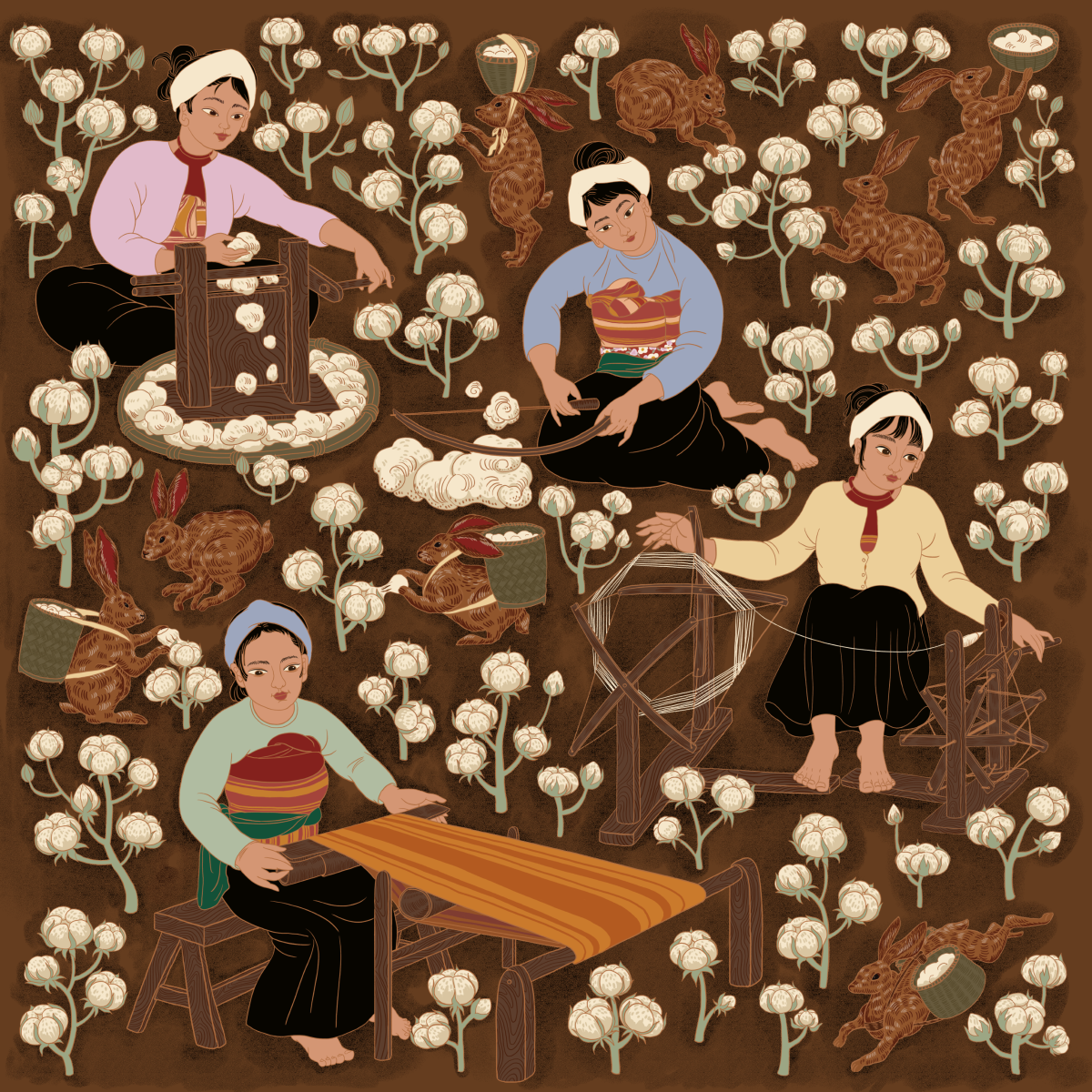The detailed painting is a square-shaped artwork with a brown background featuring four animated women engaging in various textile activities amidst a lovely scene dotted with cotton, white flower petals, and a few bunny rabbits. In the upper left corner, a woman dressed in a pink sweater with a red shirt underneath, a white headband, and black pants is depicted feeding cotton through a machine. Adjacent to her on the upper right, another woman, adorned with a white headband, a blue shirt, a red top tied around her chest, a green belt, and a black skirt, is seated and appears to be processing cotton with a bow-like tool. To her right, a third woman, also wearing a white headband paired with a yellow sweater over a red shirt and a black skirt, is threading string through what looks like a machine. On the bottom left, a woman with a blue headband, a green shirt, a red top knotted around her chest, a green belt, and a black skirt, is seated on a bench, working on what seems to be an orange blanket stretched with a wooden tool. The bright and clear setting of the painting is enhanced by natural light, giving the entire composition a vibrant and lively atmosphere.